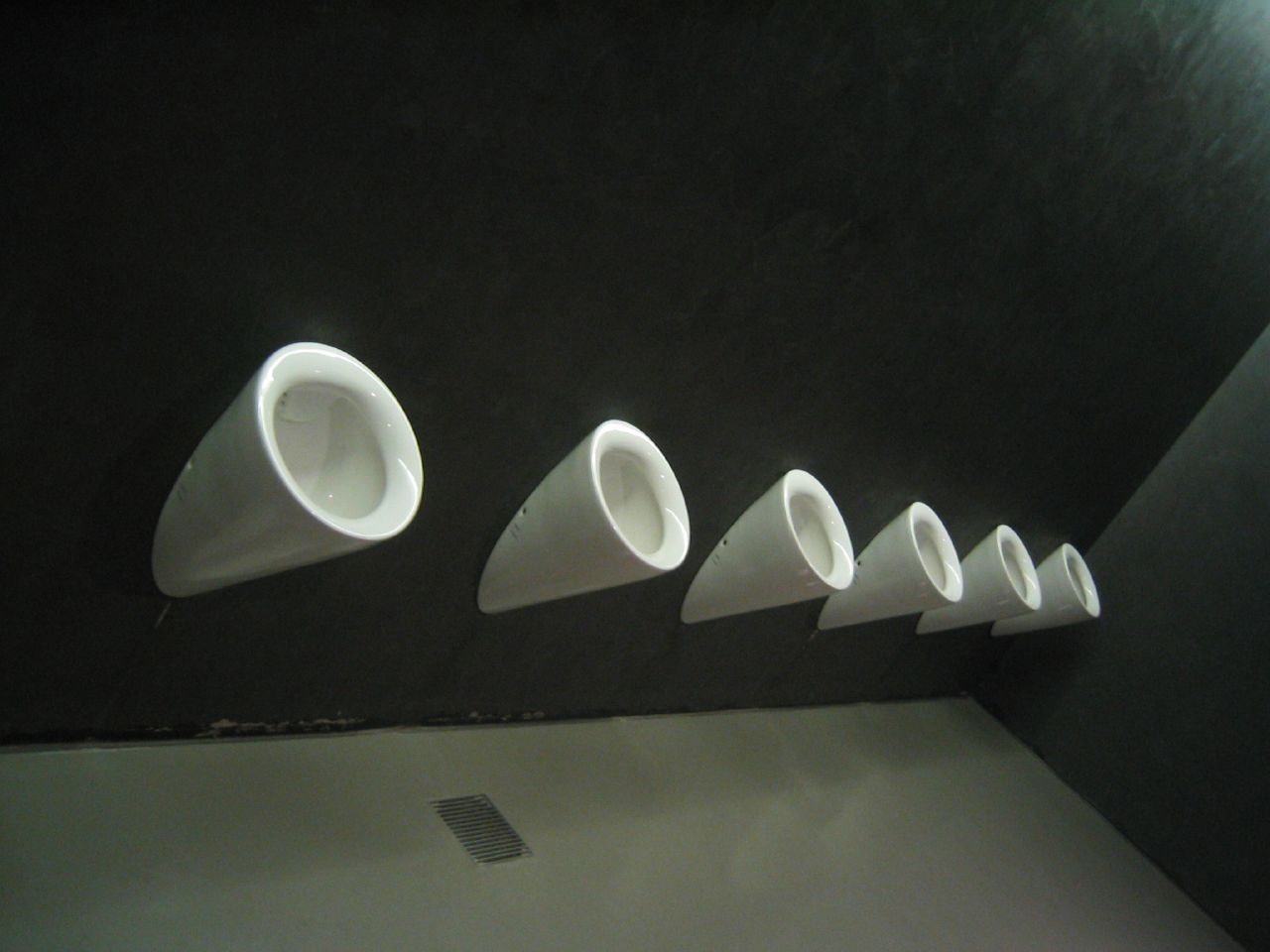The image features a series of cylindrical white porcelain urinals, artistically mounted at an angle on a sleek black wall. Each urinal has a thick rim leading into an opening, and there appears to be a mounting screw on the left-hand side of each mount. Due to the lighting from the top right corner, the adjacent wall appears darker gray in the image. The floor beneath the urinals is white, and there is some form of small object, possibly a cell phone with a cover or a grate, in view. The urinals, devoid of visible flushing mechanisms, present a modern, minimalist aesthetic. As the image progresses from left to right, the angles of the urinals become sharper, making their interiors less visible. The overall scene is both functional and visually intriguing, combining practical elements with a touch of artistic design.